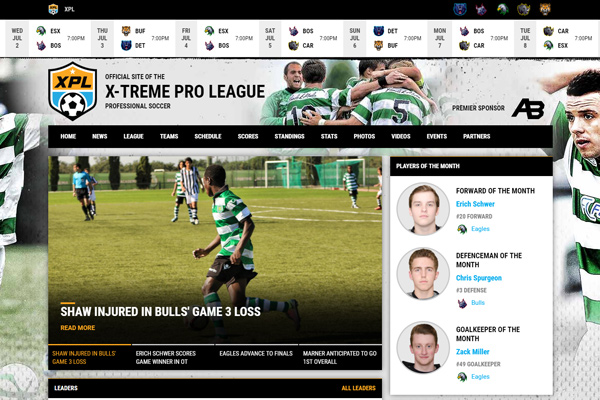This image is a screenshot of a soccer-themed website for the Extreme Pro League (XPL). The website features a prominent shield logo at the top emblazoned with "XPL" and a soccer ball at the bottom. Beneath the logo, the full name of the league, "Extreme Pro League," is clearly displayed. The visual design includes images of players dressed in striped jerseys with alternating green and white horizontal stripes, resembling short-sleeve polo shirts.

At the center of the webpage, there is a current news article headlined "Shaw Injured in Bulls' Game Three Loss." 

On the right-hand sidebar, the "Players of the Month" section highlights three standout athletes:
1. **Forward of the Month:** Erich Schwerer from the Eagles.
2. **Defensive Player of the Month:** Chris Spurgeon from the Bulls.
3. **Goalkeeper of the Month:** Zach Miller from the Eagles.

The sidebar also shows images of these players, with various other pictures depicting team members huddling and embracing in celebration. The layout is designed to provide a comprehensive overview of league highlights and top performers.